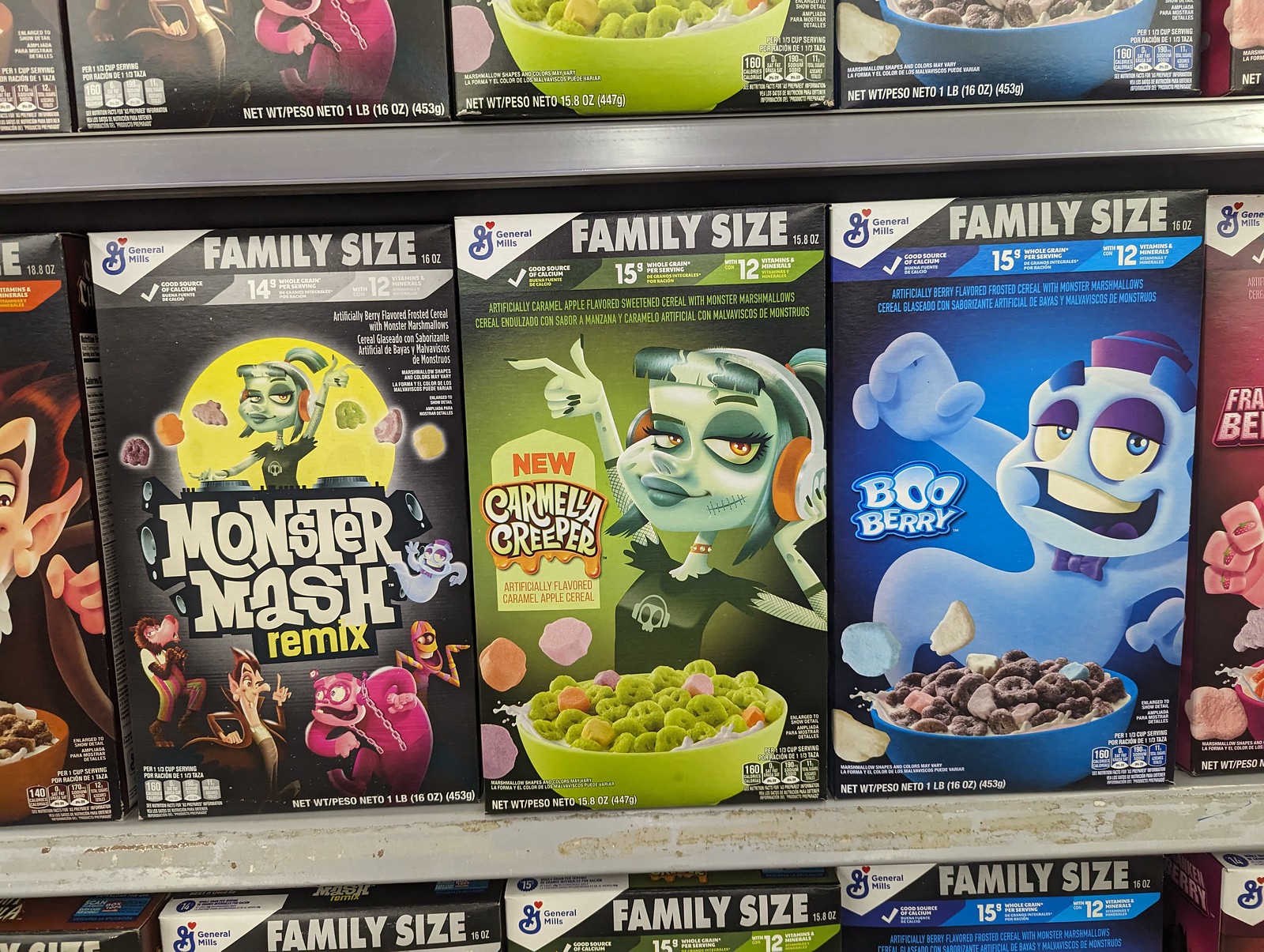The photograph showcases an up-close view of the cereal shelves in a grocery store, specifically featuring the General Mills Monster Series. Prominently displayed are family-sized boxes of Monster Mash Remix, Carmella Creeper, and Boo Berry, each adorned with vibrant and spooky thematic designs. 

Starting from the left, there's a partially visible box of Count Chocula cereal, followed by the black box of Monster Mash Remix. This box features Carmella Creeper, depicted as a green-skinned DJ with headphones, turntables, and moonlight behind her. Below her, iconic characters such as the werewolf, Count Chocula, Frankenberry, the mummy, and a ghost are depicted dancing. In the center, the green box of Carmella Creeper cereal stands out with a larger image of Carmella Creeper herself, complete with scars on her cheeks, holding a bowl of green cereal with marshmallows. To the right, the blue box of Boo Berry cereal presents a drowsy-looking blue ghost wearing a purple hat, over a bowl of blue-colored cereal with ghost-shaped marshmallows. 

On the far right, a portion of the pink Frankenberry box is visible. The shelving also shows evidence of wear with remnants of old stickers. The image highlights three tiers of these cereals, emphasizing the large quantity available. Each box features the General Mills logo and "Family Size" text at the top, along with Nutritional Facts sections. The color palette across the boxes includes shades of black, green, blue, pink, and partial visibility of brown and red, reflecting the playful and eerie redesign of these classic cereals.